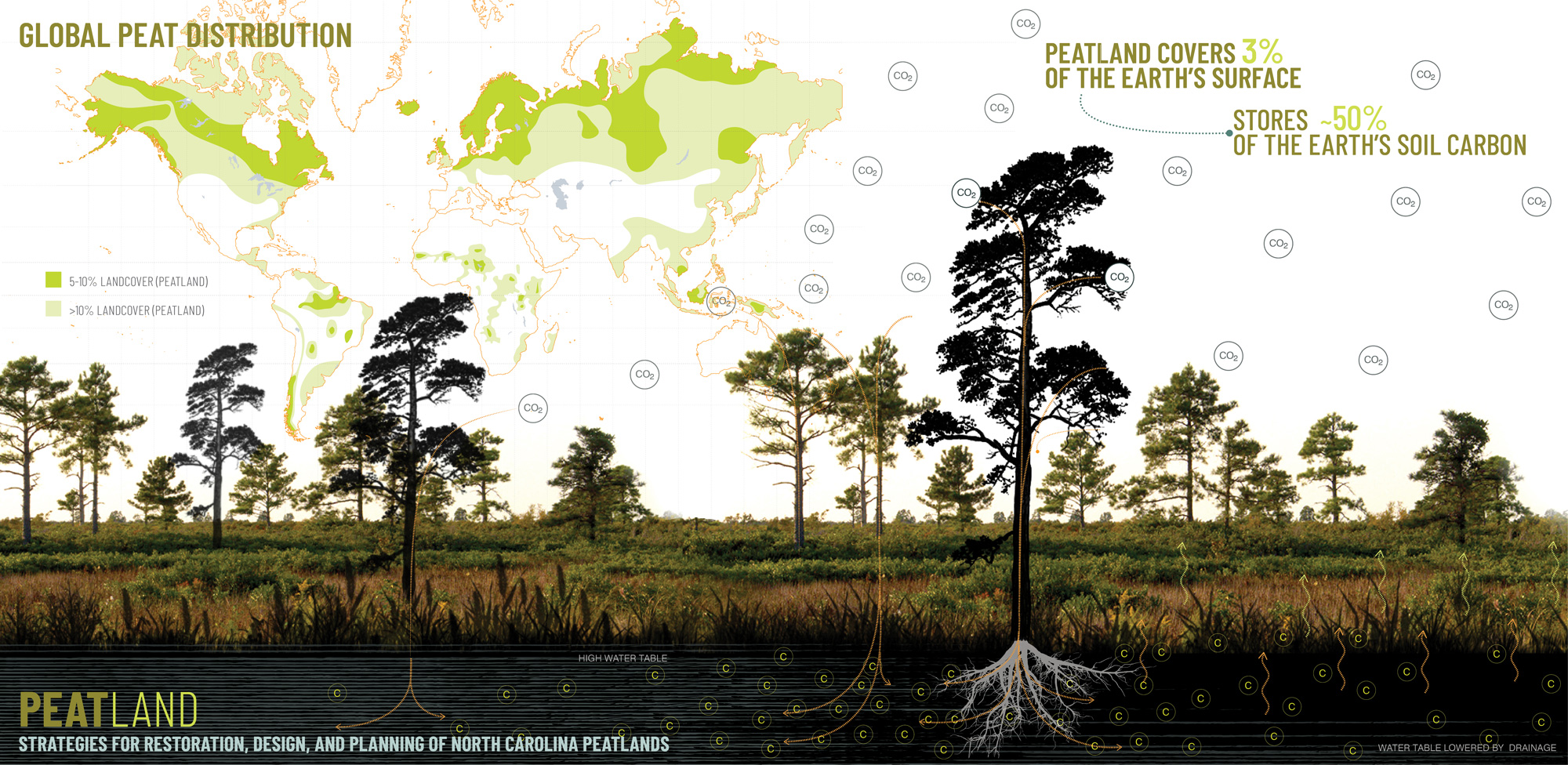The image is a detailed infographic focused on peatland conservation and restoration. At the top left, it features green text reading "Global Peat Distribution." Below this, there's a world map shaded in varying intensities of green, with a legend indicating areas covered by peatland (dark green for 5-10% land cover and light green for greater than 10% land cover). Adjacent to this, in the top right, green text highlights pivotal statistics: "Peatland covers 3% of Earth's surface, stores 50% of Earth's soil carbon." The image includes clear visual elements, showing lush green trees with visible root systems extending into the ground, emphasizing the depth and importance of root structures. Little gray circles labeled "CO2" float in the illustrated sky, illustrating the carbon absorption capability of peatlands. Additionally, there are small green circles labeled "C" beneath the ground, with wavy arrows pointing upward, symbolizing carbon sequestration. In the bottom left corner, green and yellow text reads "Peatland," with white text beneath stating "Strategies for restoration, design, and planning of North Carolina peatlands." The infographic includes a bright and clear setting with no other discernible objects or people, making it an informative and visually comprehensible piece about the importance of peatland ecosystems in mitigating climate change.